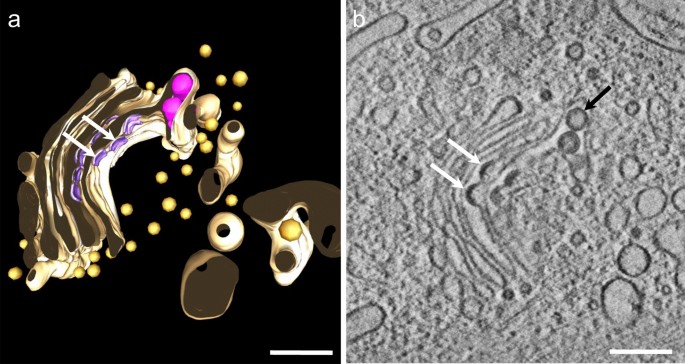This diptych showcases two images labeled A and B, potentially captured using a high-powered microscope or prepared from microscopic data. In Image A, set against a black background, we observe an intricate, colorful depiction of molecular structures. Various yellow dots, pink and purple segments, and cream, brown, and white curved lines are dispersed across the field. Two arrows point towards a prominent purple section of the molecular composition. Image B, situated to the right, offers a grayscale view of the same structures seen in Image A. Though devoid of color, the black-and-white depiction clearly identifies the abstract shapes, corresponding to the colorful features in Image A, with arrows indicating matching parts between the two images. This seamless comparison highlights how the vibrant molecular details translate into a more conventional, monochromatic microscopic image.